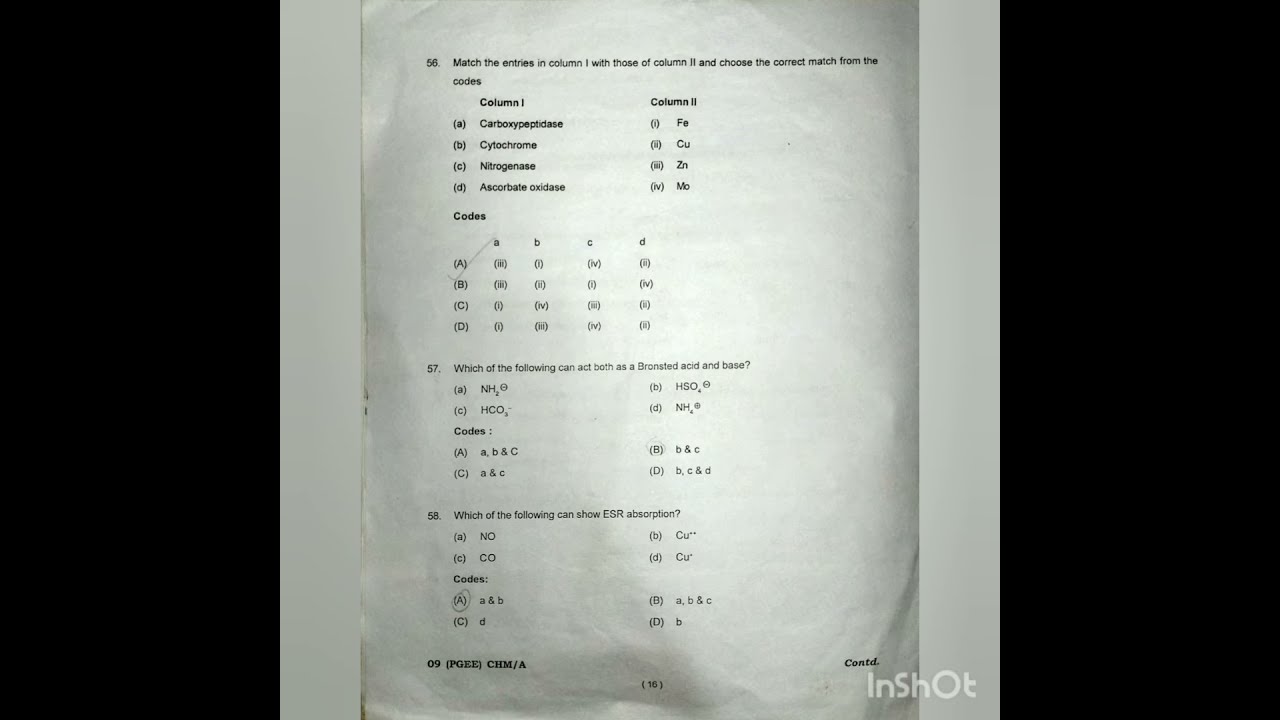This detailed image depicts a color photograph of a black-and-white exam or test page, likely related to science and chemistry, given the references to tables, graphs, and chemical symbols. The test page, centered against a white background framed by vertical black bars, contains detailed questions like matching entries between two columns (Column 1 and Column 2), with instructions to select the correct match from given codes. Notably, question numbers 56, 57, and 58 are visible, reinforcing its academic context. The page is marked at the bottom with the page number "16" in parentheses, indicating its position within a larger document. Additionally, a distinct watermark appears in the bottom right corner, reading "InShot" in a stylized format with uppercase I, N, S, H, and T, and a larger font size for the "O," pointing to the involvement of the InShot application in capturing or editing the image. The overall presentation suggests a meticulously arranged examination page, reproduced with photographic precision.